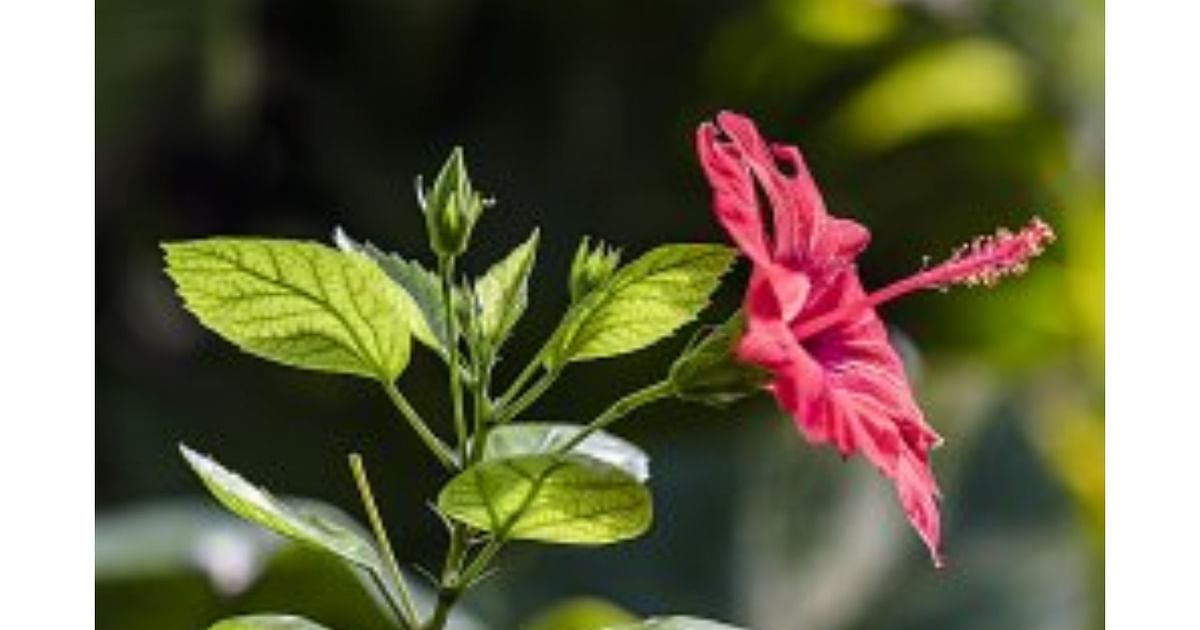In the center of the image stands a flowering plant. The focus is on a vibrant reddish-pink hibiscus bloom, which faces towards the right. This striking flower has petals radiating from its core and a prominent stamen extending to the upper right, ending in yellow filaments. Emerging from a thin green branch, this flower captures the eye, while the branch itself shoots up gracefully, adorned with delicate, almost translucent light green leaves with visible darker green veins. At the top of the plant, there's an unopened bud, displaying a darker green hue with light green triangular markings.

The background of the photograph is heavily blurred, resulting in a strong depth of field effect that renders the surroundings into indistinct patches of black, light green, and dark green hues. Sunlight highlights parts of the leaves, imparting a yellowish tinge, and the entire scene exudes a natural, serene ambiance despite the image's low quality and overall blurriness. The plant’s detailed and focused foreground contrasts with the impressionistic blur of the background, emphasizing the vivid, blooming hibiscus as the image's focal point.